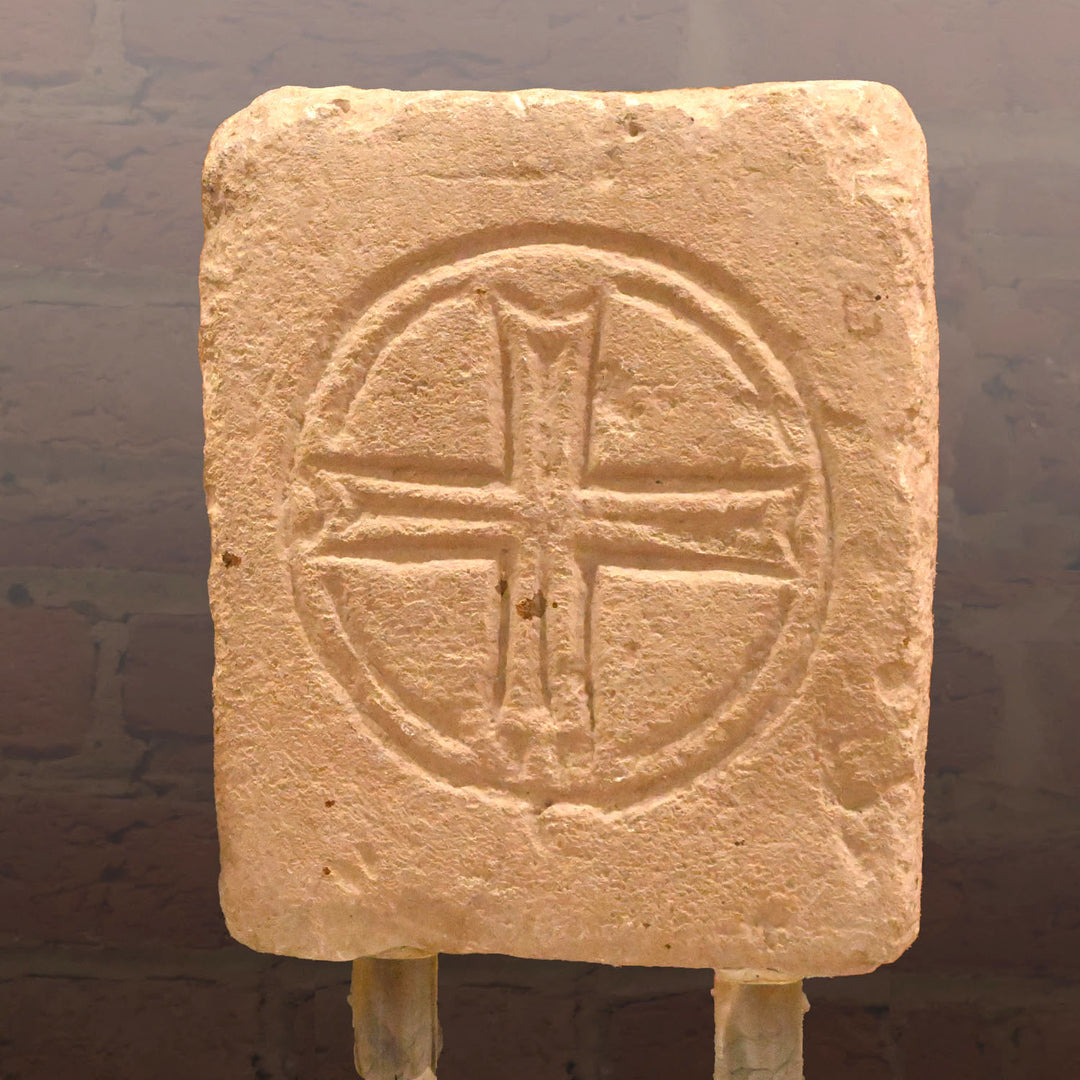The image depicts a museum exhibit featuring a weathered, square stone sculpture with a reddish hue. The stone, possibly made of limestone or cement, is intricately carved with an old, simple cross at its center, encircled by a large, etched ring. The cross resembles a basic, non-religious design, reminiscent of a symbol for organizations like Blue Cross Blue Shield. The aged stone slab, standing upright with the help of two metal or wooden sticks, shows significant imperfections, indicating its antiquity. The backdrop consists of an out-of-focus grayish brick wall, adding to the historical and rustic ambiance of the scene.